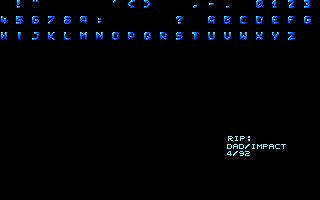This is a horizontal, rectangular color photograph depicting an old word processor computer screen. The screen, which features a black background, displays bright blue alphanumeric characters along the top three lines. The top line begins with various punctuation marks including an exclamation point, followed by the numbers 0, 1, 2, 3. The second line features the numbers 4 through 9, followed by a colon, a question mark, and then the letters A through G. The third line continues with the letters H through Z. In the lower right-hand corner of the screen, there are three lines of plain aqua text: the first line reads "RIP:," the second line reads "dad/impact," and the third line reads "4/92."